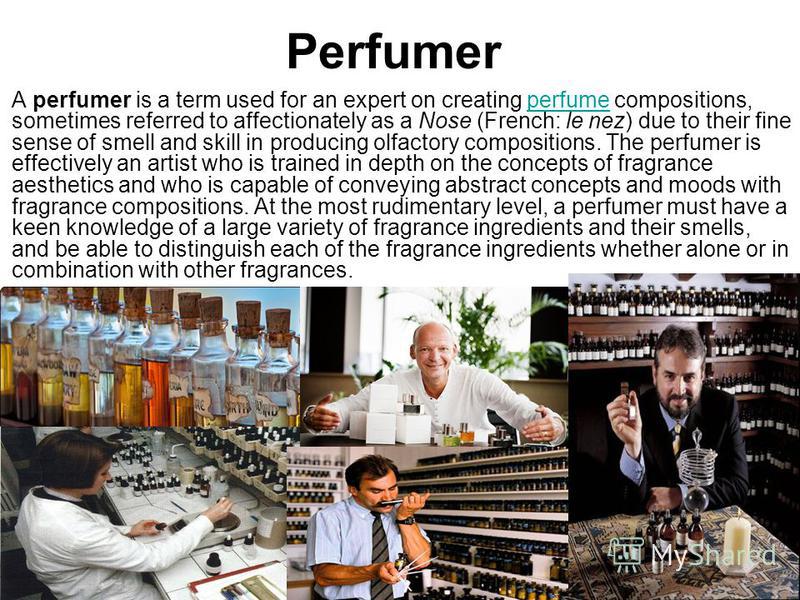This detailed image features several perfumers, each dedicated to the art and science of creating exquisite fragrance compositions. At the top of the image, the word "Perfumer" is displayed prominently in a clean, sans serif font. Accompanying the striking visuals is an informative paragraph explaining that a perfumer, often referred to as a "nose" (or "le nez" in French), is an expert in the field of perfume creation. These skilled artists possess an exceptional sense of smell and are adept at crafting olfactory compositions that evoke abstract concepts and moods. 

The text emphasizes the depth of training a perfumer undergoes, encompassing the principles of fragrance aesthetics and a vast knowledge of various fragrance ingredients. A perfumer must be proficient in identifying and differentiating the complexities of each ingredient, whether in isolation or when blended with others. The images in the composition showcase multiple perfumers in their element, highlighting their meticulous work and dedication to the nuanced world of fragrance creation.